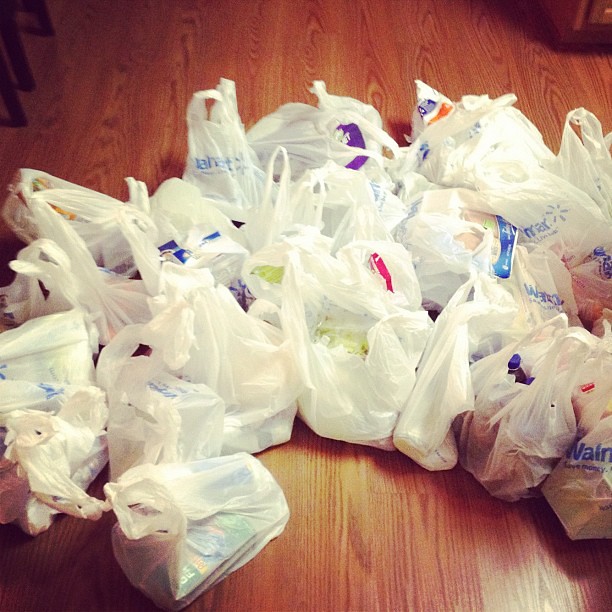The photograph captures an interior scene of someone's home, with a clear focus on the floor, which appears to be made of vertically grained brown wood, likely red oak or mahogany. In the center of the floor is a disorderly array of over 20 white plastic grocery bags, all branded with the blue Walmart logo, some of which are taped shut with blue tape. The bags are slightly translucent, suggesting they contain groceries, but the exact items are indiscernible. Hints of potential contents, like fruits and vegetables, are visible through the plastic. Additional context clues, like the outline of a dining room chair in the top left corner and an ambiguous stand in the top right, situate the scene in what might be a dining room. The setup suggests the groceries were recently delivered and placed on the floor in a casual, unorganized manner awaiting further sorting.